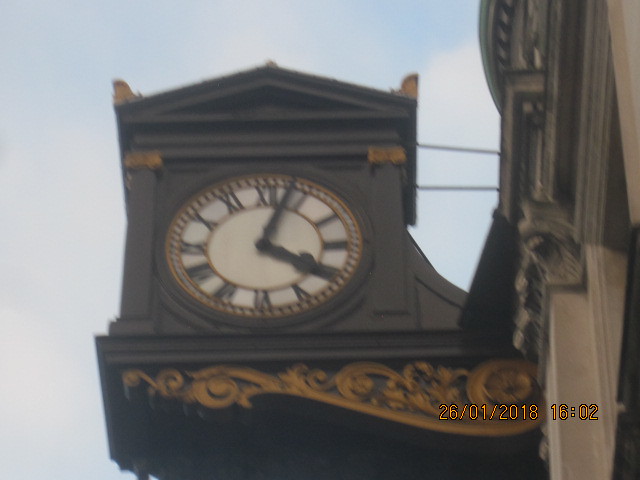This photograph, timestamped in orange at the bottom with "26-01-2018" and "16:02," showcases an intricate, old-fashioned clock mounted high on the side of a tan-colored building. The clock, secured by two thin metal posts, features a dark chocolate brown body adorned with gold leaf details. Its pale tan clock face is elegantly marked with dark brown Roman numerals and matching hands, all encased by a gold circular decorative pattern along the edge. Beneath the clock face, the dark brown body continues, embellished with elaborate gold carvings that enhance its ornate appearance. To the left side of the image, a portion of the building with bronze-colored carvings is also visible, adding to the historical and artistic feel of the scene.